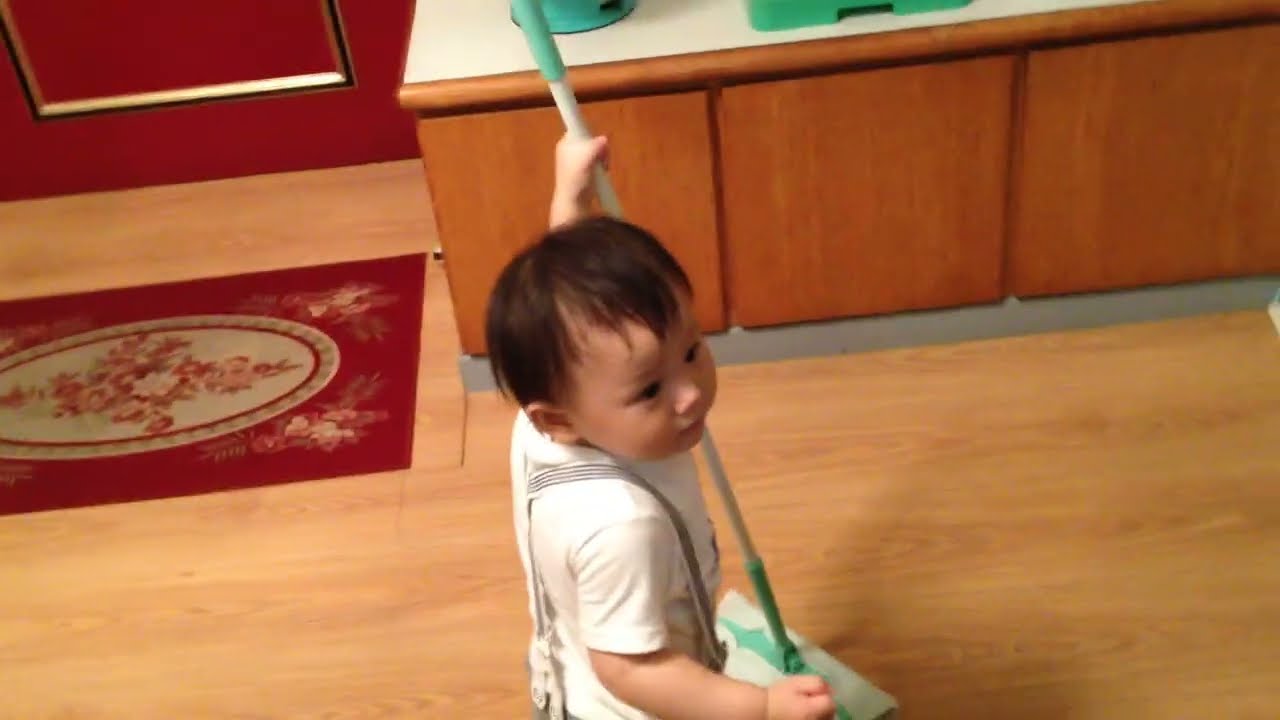A young Asian boy, approximately three years old, stands in what appears to be a kitchen, adorned in a white short-sleeved shirt and black suspenders holding up shorts or pants. His dark hair frames his face as he looks up toward the camera, which is likely being held by the person capturing the moment. He wields a Swiffer mop with an aqua handle and base. The scene is set on a light wooden laminate floor, accentuated by a distinctive red rug with a floral pattern in front of a door featuring a gold trim and a rectangular design at its base. Behind him are three closed cabinet doors with golden brown fronts and a white countertop that aligns with his height, further defining the indoor setting.